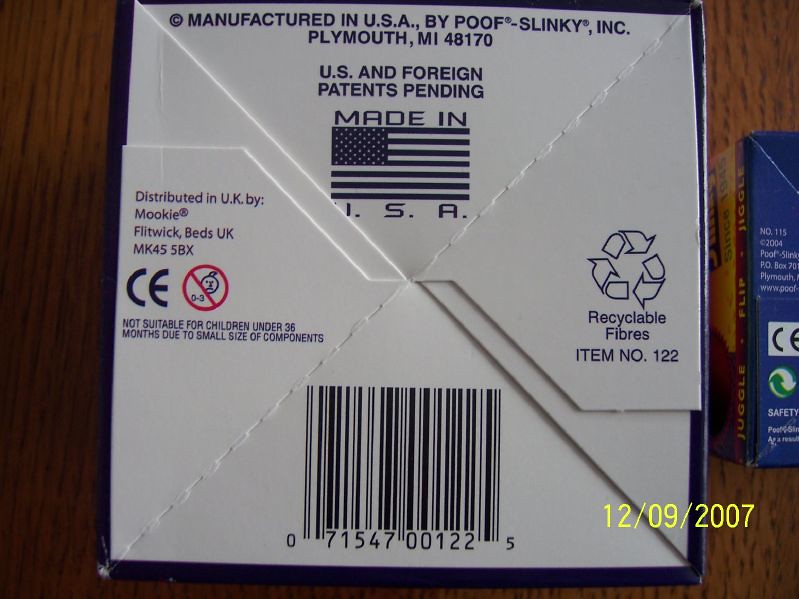This is a photograph in a slightly rectangular format with a width greater than its height. At the bottom of the image, there is a yellow date stamp indicating "12-09-2007," suggesting that it is an older photo. The foreground features a wood grain desk, which covers the bottom part of the image. 

The main subject of the photograph is a partially visible product box, predominantly showing the underside. The text on the box reads: "Manufactured in USA by Poof Slinky Incorporated, Plymouth, Michigan, MI 48170. U.S. and foreign patents pending, made in USA." This confirms that the product is a Slinky, a well-known classic toy. 

Additionally, the box mentions distribution details: "Distributed in UK by Mookie, Flitwick Beds UK, MK45 5BX,” indicating that this American-made Slinky is also sold in the United Kingdom. 

To the right of this box is another upside-down box that reads "jiggle, flip, and wiggle" on its side, suggesting it contains another classic childhood toy, possibly Play-Doh or something similar.